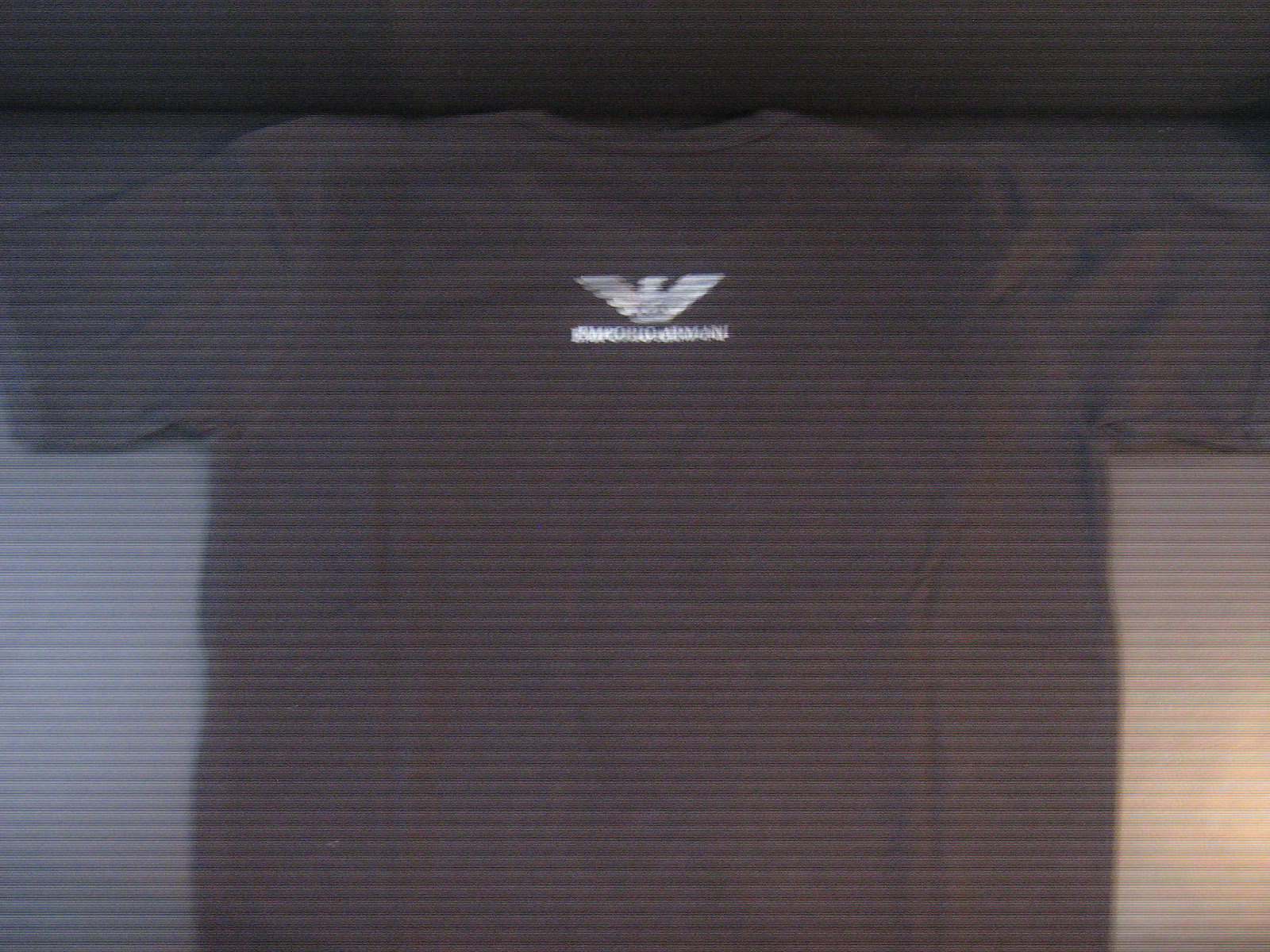This indoor, close-up color photograph features a gray t-shirt lying flat on a surface. The shirt exhibits a distinct horizontal lining in its fabric, creating a subtle pattern extending from the top to the bottom. Positioned near the neck on the upper portion of the t-shirt is a white emblem resembling a "V" with an additional symbol in the center, although it's difficult to discern due to the slight blurriness of the image. Beneath this emblem, the letters "R P O R I O" can be seen, followed to the right by "A R M A N I". This suggests that the t-shirt is likely branded. The shirt's fabric appears slightly lighter in the right corner of the photograph, and there are white segments in both the lower left and right corners, adding a unique visual contrast to the predominantly gray garment.